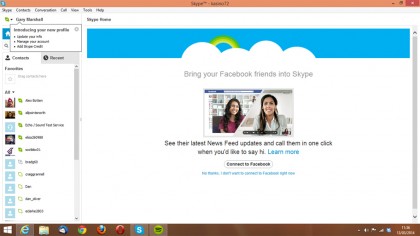This screenshot captures a promotional feature of Skype, highlighting the ability to integrate Facebook friends into the platform. Dominating the center of the image is a prominent message: "Bring your Facebook friends into Skype." To the left, there is a vertical menu characteristic of the Skype interface.

In the main section, two women appear to be on a video call. The woman on the left has black hair and is wearing a short-sleeved purple top. She is sitting down, with a brown chair visible behind her. The woman on the right also has black hair and is dressed in a white top. Below this visual representation of the call, text reads: "See their latest news feed updates and call them in one click," followed by an invitation to "learn more" through a hyperlink.